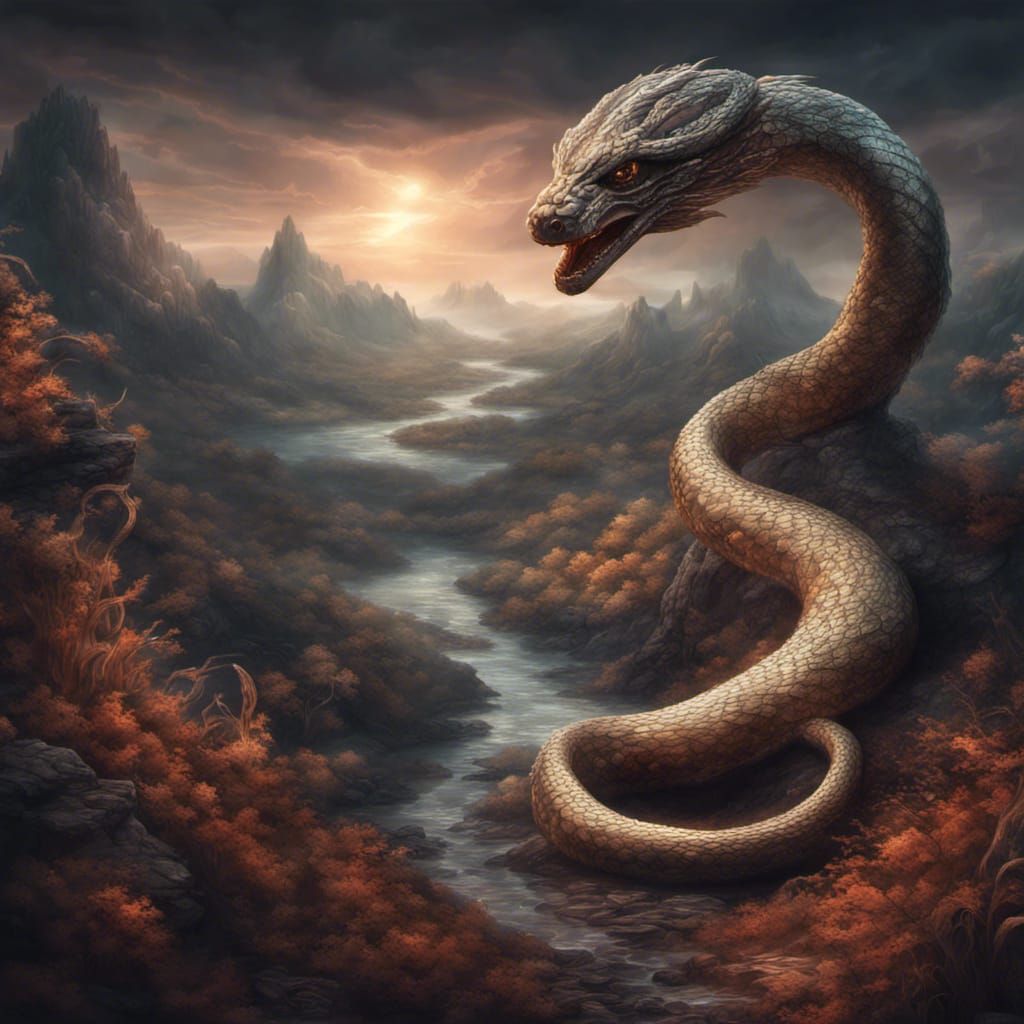This computer-generated fantasy illustration depicts a colossal, serpentine dragon dominating a jagged, mountainous valley. The dragon, positioned toward the right side of the image, coils ominously around a meandering, blue-grey stream that cuts through the rugged landscape. Its fierce golden eye gleams as its mouth, tinged with red, opens wide, ready to unleash its fury upon the valley's sparse and rugged foliage. The scene is enveloped in a stormy atmosphere, with dark, brooding clouds overhead, and the sun struggling to peek through, casting a dramatic light upon the dragon's grey scales. The entire composition has a surreal, fantastical quality akin to scenes from epic tales like "The Lord of the Rings," marked by an eerie, reddish tint that heightens the ominous and otherworldly undertones of the ravine.